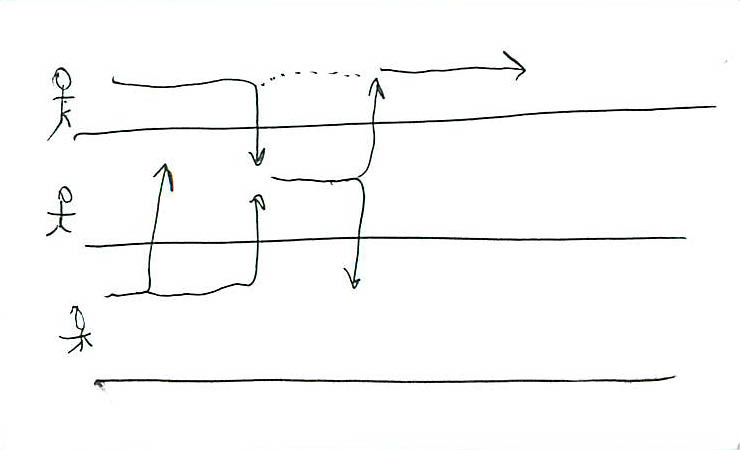A roughly sketched illustration features three simplistic stick figures set against a faint gray box background. At first glance, the white screen background appears dominant, but closer inspection reveals a subtle gray rectangular enclosure framing the figures. Each stick figure, devoid of facial features and details, is depicted in minimalistic black lines that resemble a photocopy.

In the first segment, the stick figure extends a black line horizontally to the edge of the encompassing box. This line branches into a downward arrow and an upward-dashed arrow, indicating multiple directions. To the right of the dashed line, another straight line with an arrow is drawn.

The second stick figure, positioned directly below the first, is similarly rudimentary, accompanied by a long black line sprouting arrows in various directions, different from those in the first segment.

Finally, the third stick figure, placed beneath the second, features a straightforward black line without any directional arrows. The simplicity and repetition of the rough lines and stick figures suggest a conceptual representation or an instructional diagram.